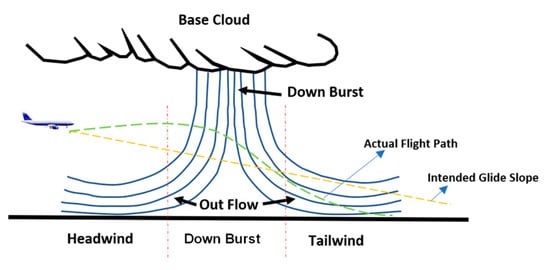The image is a detailed black and white diagram, reminiscent of a figure from a science textbook, displayed against a white background. At the top, a labeled "base cloud" is illustrated with black and white drawings of a cloud. Below the cloud, multiple lines extend downwards, some angling left and others right, annotated as a "downburst" with arrows indicating the direction of air or water. Blue lines further illustrate the downburst, showing the flow direction. An airplane, depicted in dark blue, is seen with its flight path marked by dotted lines, intersecting these downburst lines. This intended trajectory highlights how the aircraft is affected by the weather phenomenon, detailing its deviation due to headwind, downburst, and tailwind. Additionally, the diagram includes text denoting "actual flight path" and "intended glide slope" with yellow areas emphasizing the comparison. At the bottom, the terms headwind, downburst, and tailwind are clearly labeled, providing a comprehensive visual explanation of the effects of a downburst on the airplane's flight path.